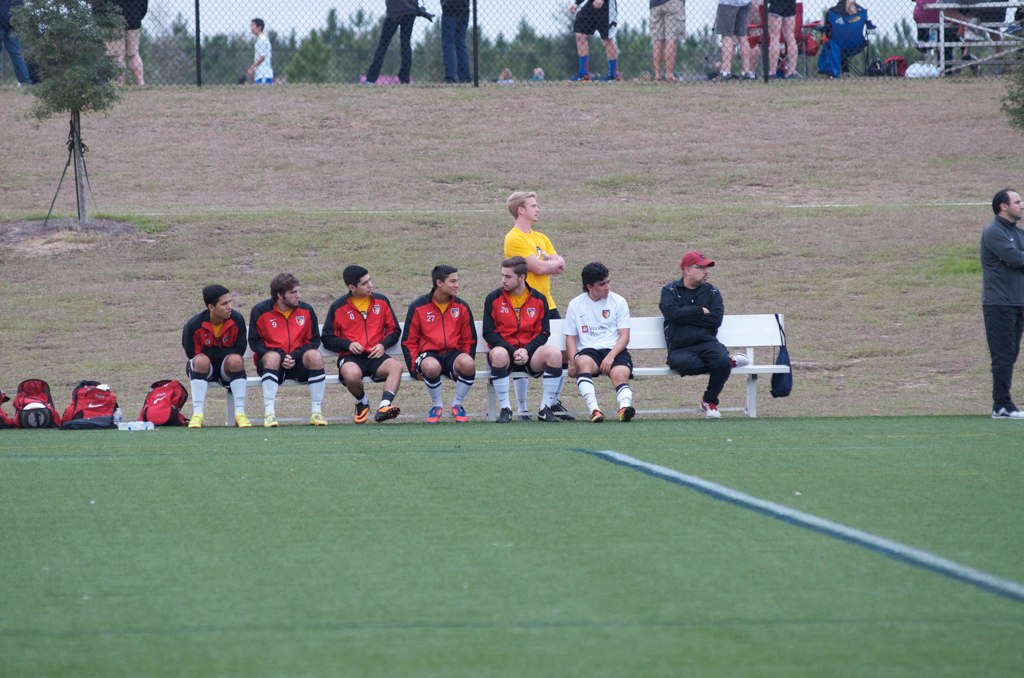The image depicts the sidelines of a soccer field where a group of men, presumably soccer players, are seated on a long white bench, likely made of fiberglass or metal. These seven players are uniformly dressed in matching black shorts and black and red jacket combinations, with white socks and athletic shoes. Over these jackets, they are wearing yellow shirts. To the left of the bench, there are three red and white backpacks on the grassy ground. Among the men, one stands behind the bench with his arms crossed, wearing a yellow t-shirt and black shorts, sporting blonde hair.

Additionally, there is a coach, distinguishable by his long black pants, a black jacket, and a red baseball cap, standing near the seated players. A black bag is hanging off the side of the bench. In front of the group is the green soccer pitch, and in the background, there's a hillside with a grayish-brownish-green hue. Behind the chain-link fence at the rear, the lower halves of spectators' bodies are visible, indicating they are watching from the other side. There is no active gameplay in sight, suggesting the players might be on a break or it is halftime.